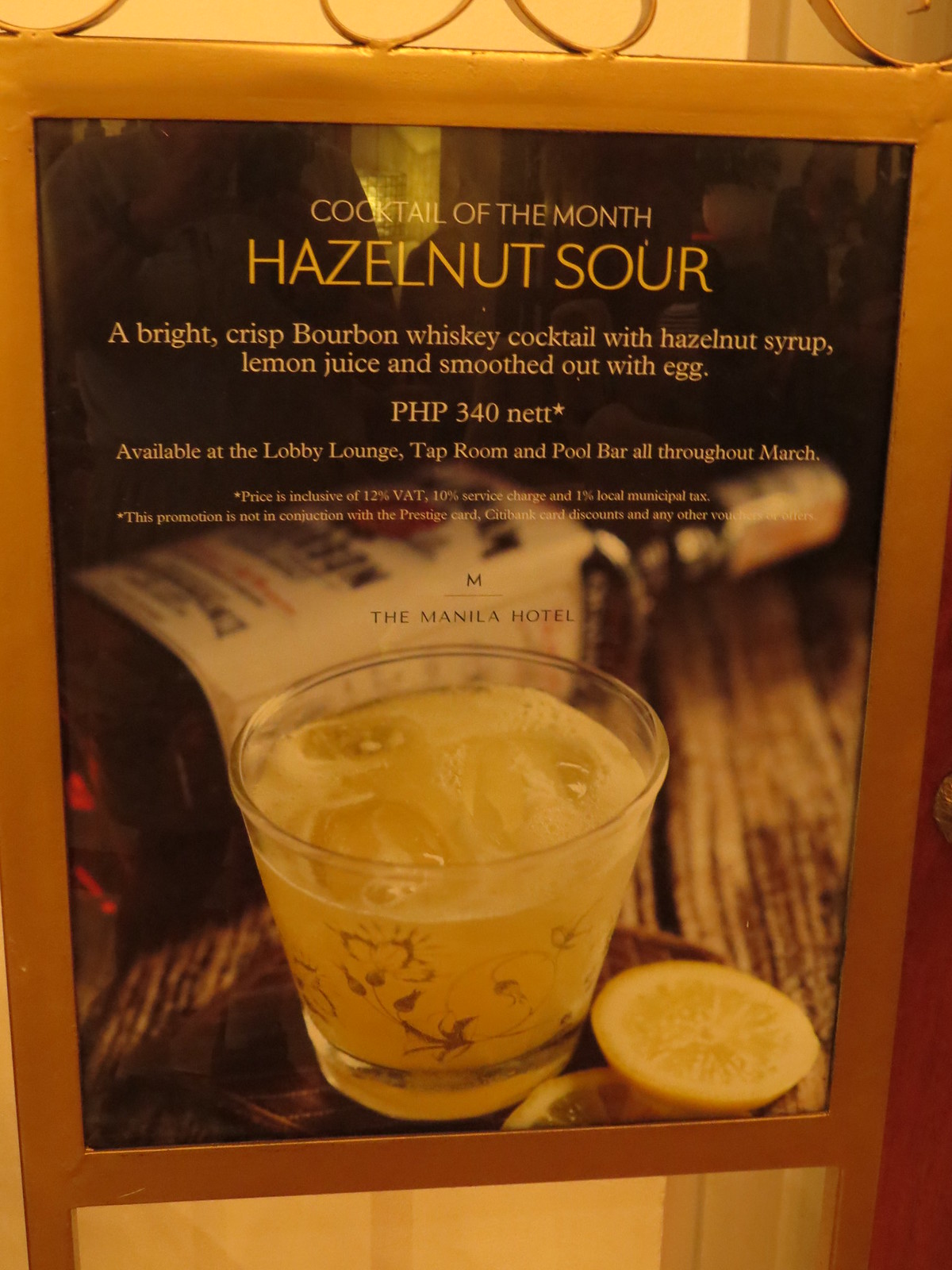The image features an advertisement for the "Cocktail of the Month" displayed on a small standing billboard encased in a metal frame. The ad promotes the "Hazelnut Sour," described as a bright, crisp bourbon whiskey cocktail mixed with hazelnut syrup, lemon juice, and smoothed out with egg, priced at PHP 340 net. The price includes a 12% VAT, 10% service charge, and 1% local municipal tax, and the promotion is not valid with the Prestige Card, Citibank card discounts, or any other offers. The drink is available at various spots within a hotel such as the Lobby Lounge, Taproom, and Pool Bar throughout March. The image has a glossy finish, reflecting the silhouettes of people nearby, and shows a filled glass of the hazelnut sour cocktail accompanied by two lemon peels and ice, sitting on a coaster. Next to the glass lies a toppled bottle of Jim Beam, enhancing the promotional aesthetics suitable for a dimly lit restaurant or hotel lounge setting.